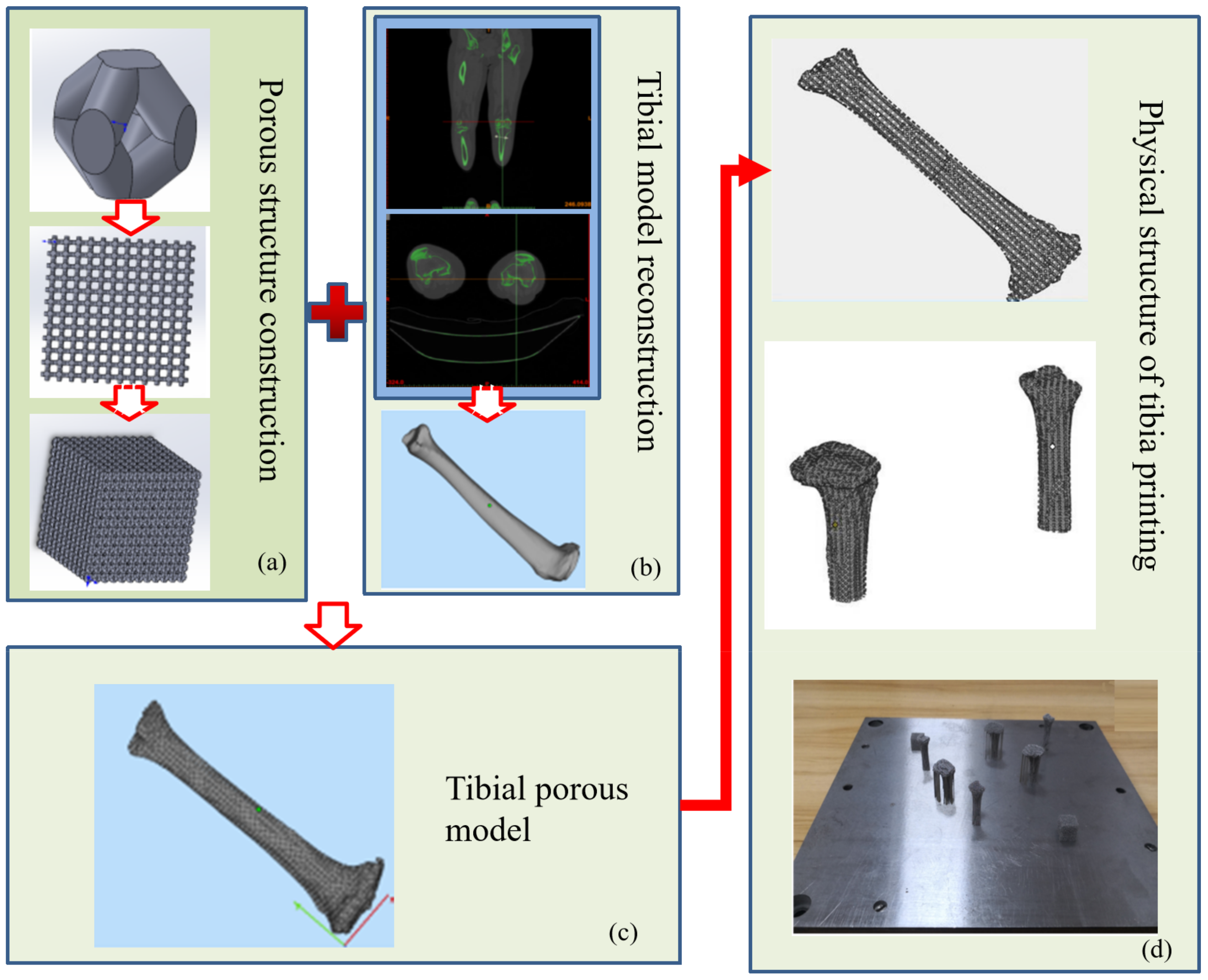The image depicts a detailed process of 3D printing a tibia bone model, emphasizing its physical structure. It features a step-by-step visual representation, including 3D-printed tibia models on small bases, and a reconstruction highlighting anatomical accuracy. There are two x-ray images showcasing different views of a tibia, illustrating its internal structure. Additionally, the image includes diagrams of porous structures and grid-patterned designs, detailing the construction phases. The final model exhibits a porous tibia design, analyzed within concentric circles, grids, and square frameworks, emphasizing the innovative aspects of the 3D printing technique used.